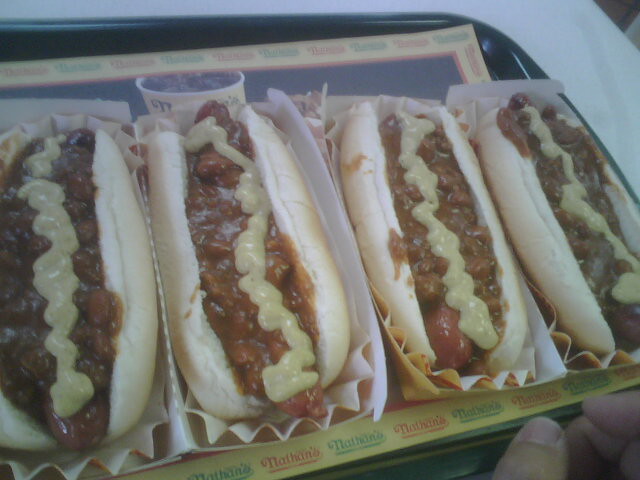This is a faded and muted color photograph taken from an angled top-down view of four chili dogs arranged side by side on a black plastic tray. Each hot dog sits in a ruffled paper liner inside a cardboard hot dog box, all positioned vertically from top to bottom within the frame. The buns are pale and simple, with a noticeable shine from the grease. The hot dogs themselves are reddish-brown, generously topped with sloppy, dark brown chili, and drizzled with a squiggly line of light yellow mustard running the length of each dog. The tray is covered with a paper placemat featuring a yellow border with the "Nathan's" logo in alternating red and green letters repeating all around. The black tray rests on a white table, and in the lower right corner of the image, a person's light-skinned thumb and index finger are visible, touching the tray's edge.